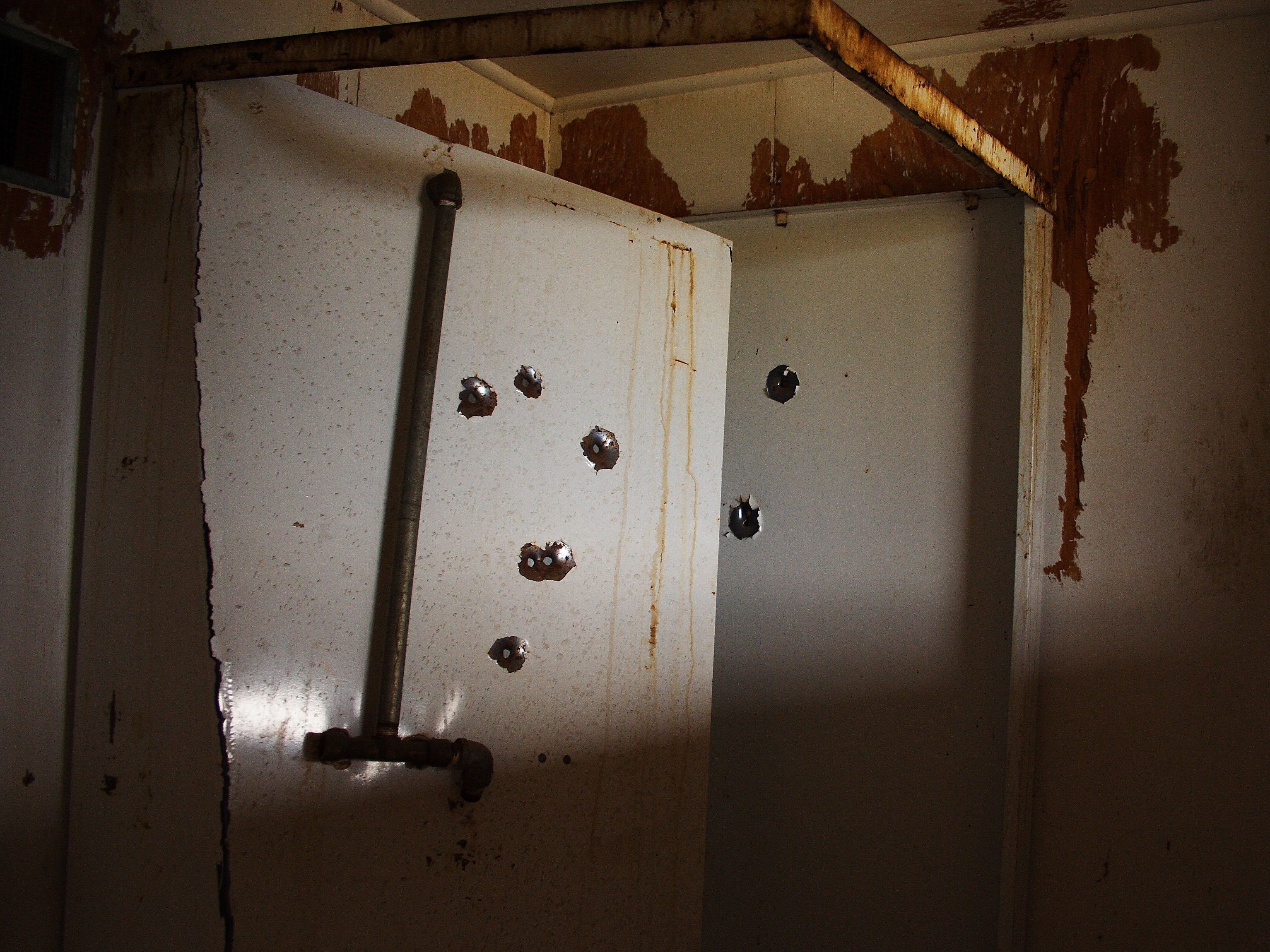This photo depicts a neglected and dilapidated room, which appears to be a basement or obscure storage area. The room is square-shaped and its intended white walls are marred by extensive peeling paint, revealing large, irregular patches of brown wood beneath. A triangular frame structure extends from the top left to the upper middle right of the photo, resembling a shower rod but with no curtain present, creating an open, yet enclosed feel to the space.

The wall within the triangular frame is heavily stained with rust-like streaks, and it houses a dark gray pipe that runs vertically before bending to a perpendicular orientation. Numerous silver bolt-like notches are visible on a white door within the frame, though their purpose remains unclear.

Another white door is part of the makeshift enclosure, featuring two gray circular holes. The entire room exudes an atmosphere of severe neglect, with rust, dirt, and decay evident throughout. This space clearly requires extensive cleaning and maintenance.